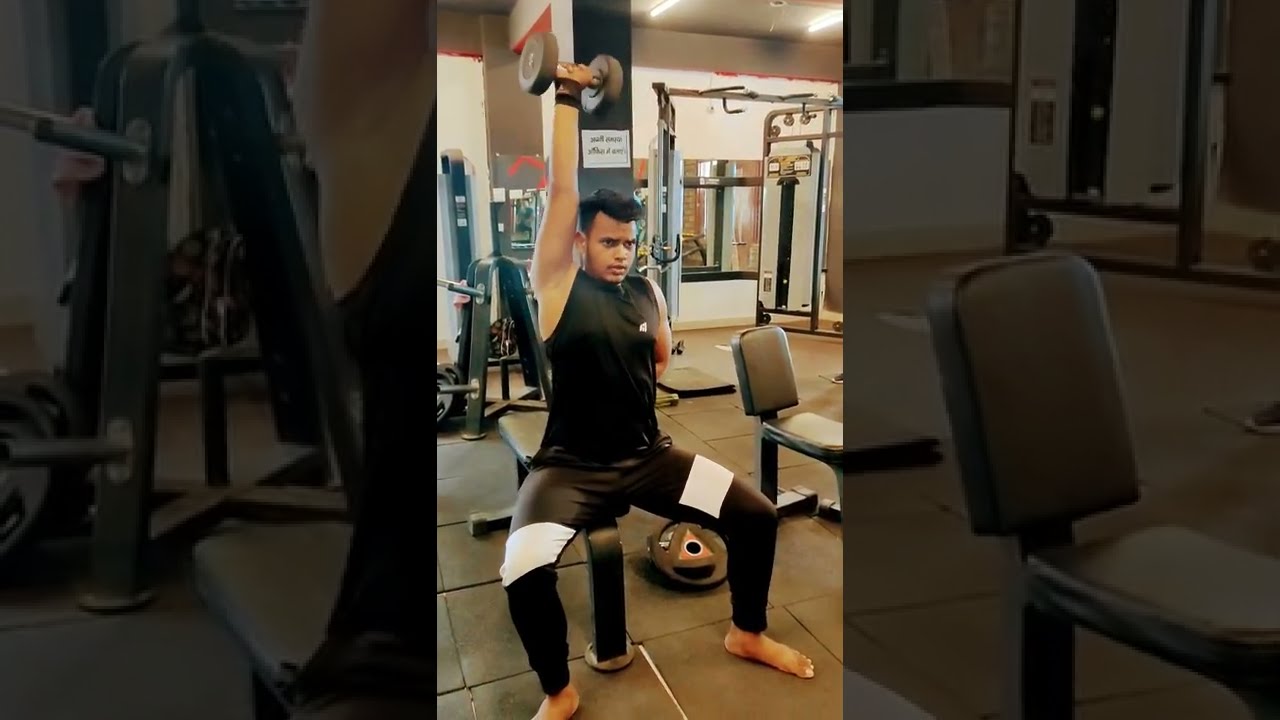This photo captures a young Indian man working out in a gym, sitting on a flat black bench while lifting a black dumbbell overhead with his right arm fully extended. He is wearing a black sleeveless shirt, black pants with white stripes on the thighs, and no shoes or socks. His left arm is obscured behind him, and he has a sweatband around his right wrist. The gym floor is covered with black foam tiles, and various workout equipment is visible in the background, including another bench to his left and a universal machine in the distance behind him. Directly behind his head, there is a black support beam. The ceiling of the gym is light gray with a red border along its length and features two ceiling lights. This image is presented in three segments: a central segment showing the man in full, a right segment zooming in on the right side showcasing another bench, and a left segment focusing on the man's right shoulder and torso with additional gym equipment in the background.